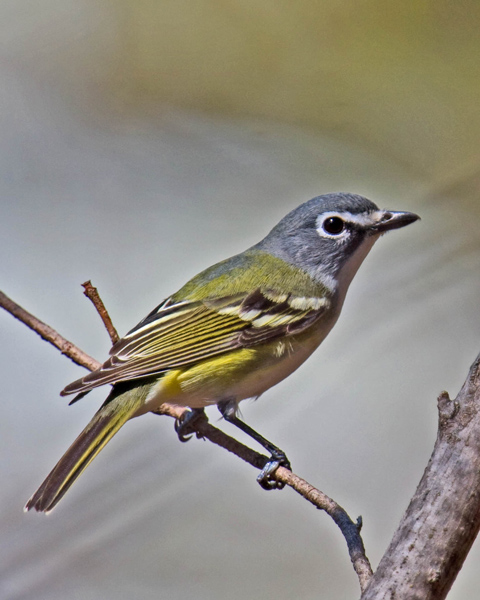This is a vertical rectangular high-resolution photograph of a small, intricately colored bird perched on a slender twig that branches off from a larger, leafless tree branch. The bird's delicate, somewhat fragile appearance is accentuated by its diverse and vibrant plumage. It boasts a striking blue head with a black eye, encircled by a subtle white ring extending towards its neutral-colored, short beak. The bird's belly is primarily yellow, blending into a whitish or pale hue, while its wings showcase a harmonized mix of brown, yellow, white, and black near the top. Flecks of green and yellow embellish its back and sides. The tail feathers display alternating green and black stripes. The bird's legs are represented as gray, and it stands out vividly against the bare, textured bark of its perch, creating an intriguing and almost surreal visual experience.